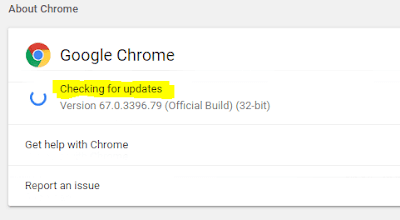This image is a screen capture of a pop-up window within the Google Chrome browser. The interface features characteristic gray borders surrounding the pop-up, with a horizontal gray bar at the top, a thinner vertical gray bar on the left, and another thinner horizontal gray bar on the right. These borders likely represent the background of the website that triggered the pop-up.

In the top left corner of the pop-up, "About Chrome" is displayed prominently in black, bolded text against the gray bar. Below this header, a white section contains additional information.

At the top left of the white section is the iconic multicolored Google Chrome logo—featuring green, yellow, red, and blue segments. To the right of the logo, "Google Chrome" is written in bold black text. Directly beneath this header is a faint horizontal gray line.

To the left, positioned below the faint gray line, is a blue letter "C," rotated 90 degrees counterclockwise, making the left side of the "C" appear at the bottom. To the right of this blue "C," text highlighted in yellow reads "Checking for updates," followed by the version number "67.0.3396.79." Additionally, the text "Official Build" and "32-bit" are displayed in black, enclosed in parentheses.

Beneath another light gray horizontal line, the bolded text "Get Help with Chrome" appears. Yet another light gray line follows, and under it, the phrase "Report an Issue" is written in black.

This detailed pop-up provides specific version information and options for obtaining help or reporting issues with the Google Chrome browser.